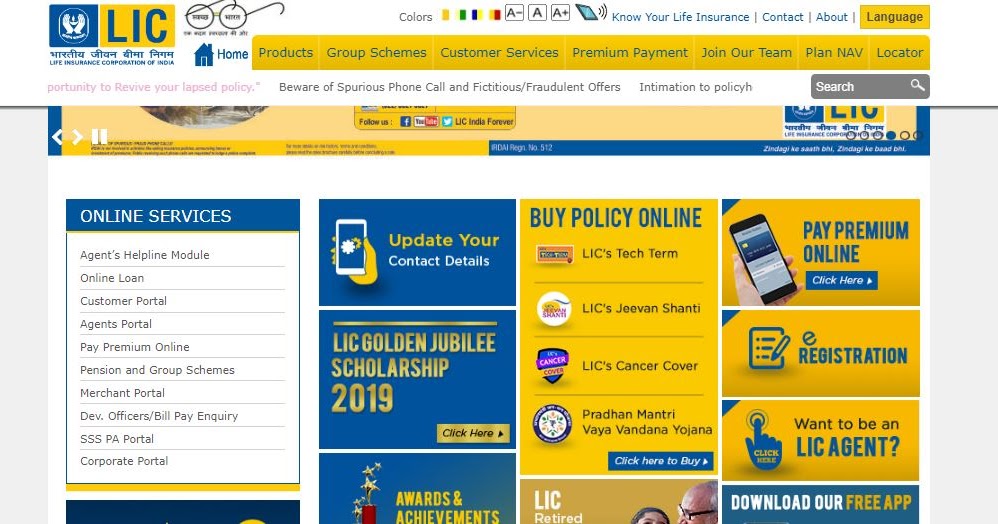The screen capture depicts the homepage of the Life Insurance Corporation of India (LIC), an Indian-based insurance company. The top-left corner prominently features the LIC logo in yellow and blue, accompanied by the full name "Life Insurance Corporation of India" written in both English and Hindi. Adjacent to the logo, a small icon of spectacles and a home tab can be seen.

A distinct yellow navigation bar stretches across the top of the page, offering various categories for user navigation, including "Products," "Group Schemes," "Customer Services," "Premium Payment," "Join Our Team," "Plan," "NAV," and "Locator." To the right of this bar lies a gray search box, facilitating easy access to specific content.

Below the navigation bar, on the left side of the webpage, a white box with blue and gold outlines is labeled "Online Services." This section includes a comprehensive list of services such as "Agent's Helpline Module," "Online Loan," "Customer Portal," "Agent's Portal," "Pay Premium Online," "Pension and Group Schemes," "Merchant Portal," "Development Officers," "Bill Pay," "SSPA Portal," and "Corporate Portal."

The main content area of the homepage is adorned with a series of blue and gold boxes. Key highlights include:
- An option to update contact details.
- Information about the 2019 Golden Jubilee Scholarship.
- A section showcasing awards and achievements.
- A central feature for purchasing policies online.

On the right side, there are additional options to pay premiums online, register, explore becoming an LIC agent, and download the free app. The website's layout is clearly designed to provide multiple entry points for users to access various services and information efficiently.